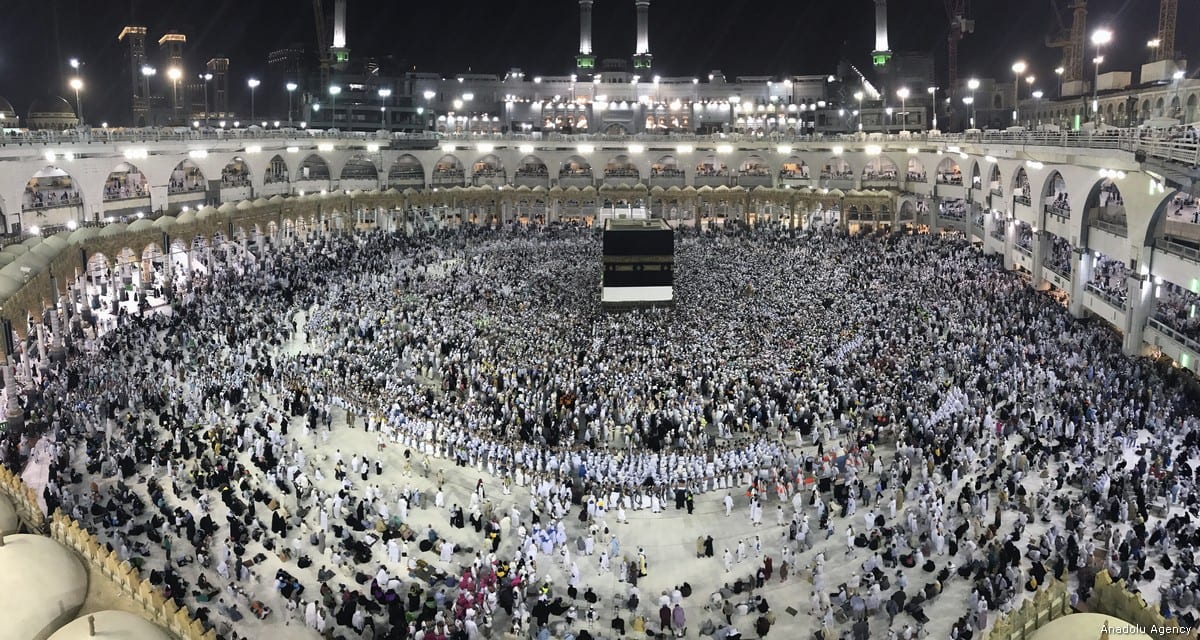This photograph captures a bustling nighttime event taking place in a massive, circular structure reminiscent of the Colosseum in Rome, though not in as good condition. The interior is illuminated with numerous lights lining the top rim and lower levels, highlighting the architectural arcs that encircle the space. The venue is packed with a sea of people, thousands of them, organized neatly across various levels and within enclosed seating areas. The central plaza, though not a traditional field, is the focal point of the gathering, featuring a large black square structure or a screen. In the background, several buildings, including a few skyscrapers and a notably large, wide building, form an urban skyline, though they are only partially visible against the night sky. This grandiose setting suggests it might be a central, important location for gatherings, possibly a nation's significant venue for public events.